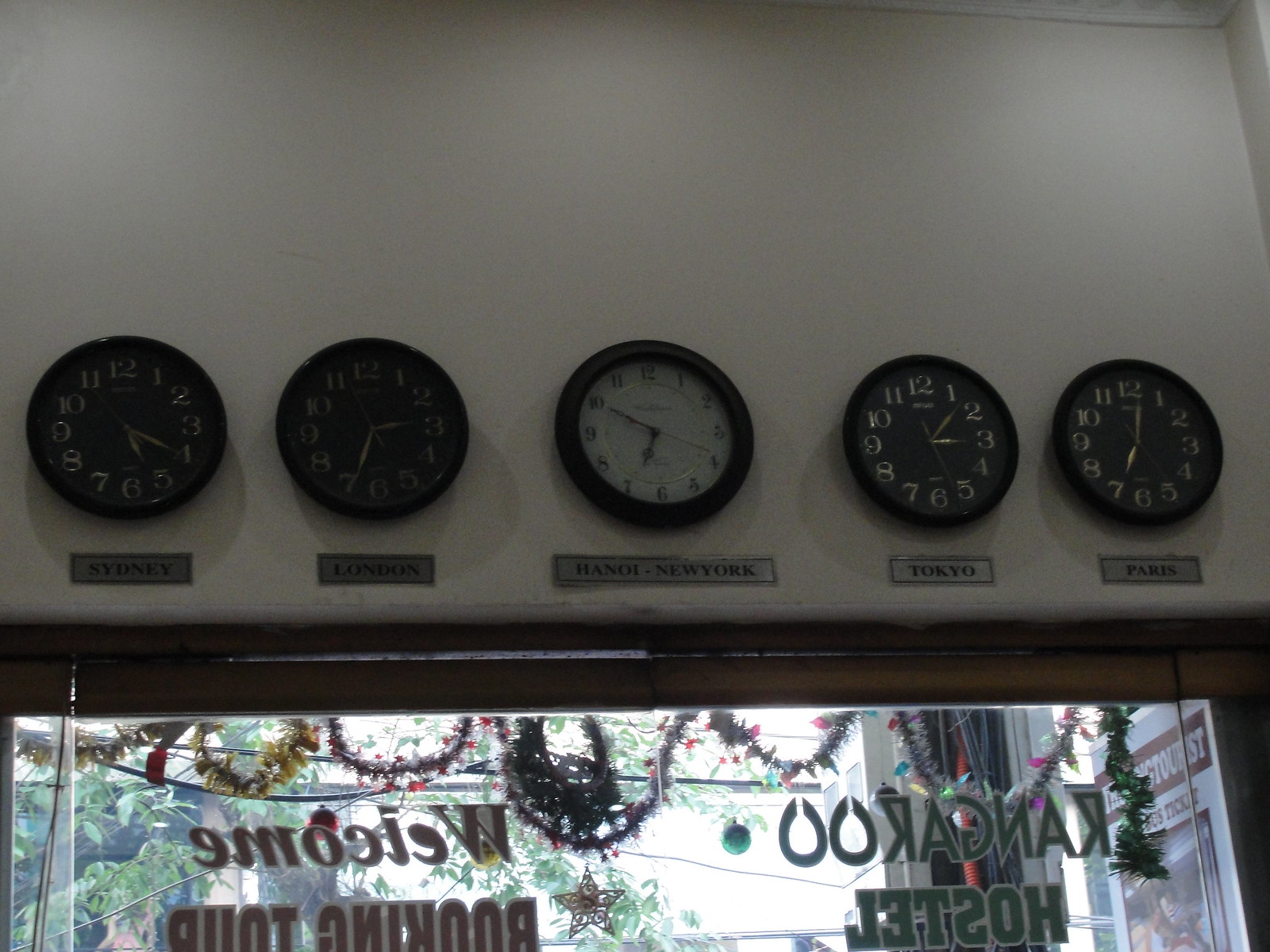A series of five clocks adorns a white wall inside a hostel room, positioned above a large window. Each clock features a dark face, with the exception of the middle one, which prominently displays the time as 10 minutes to 7. Below this central clock, a label reads "New York Time." Flanking this clock to the right, another indicates "Tokyo Time," and the one furthest to the right shows "Paris Time." The two clocks on the left are harder to decipher in terms of their time settings. Below the clocks, the window offers a view of a large tree outside. Inscribed on the inside of the glass, the words "Kangaroo Hostel" appear on the right side, while "Welcome" and "Booking" are partially readable on the left, with other text obscured.